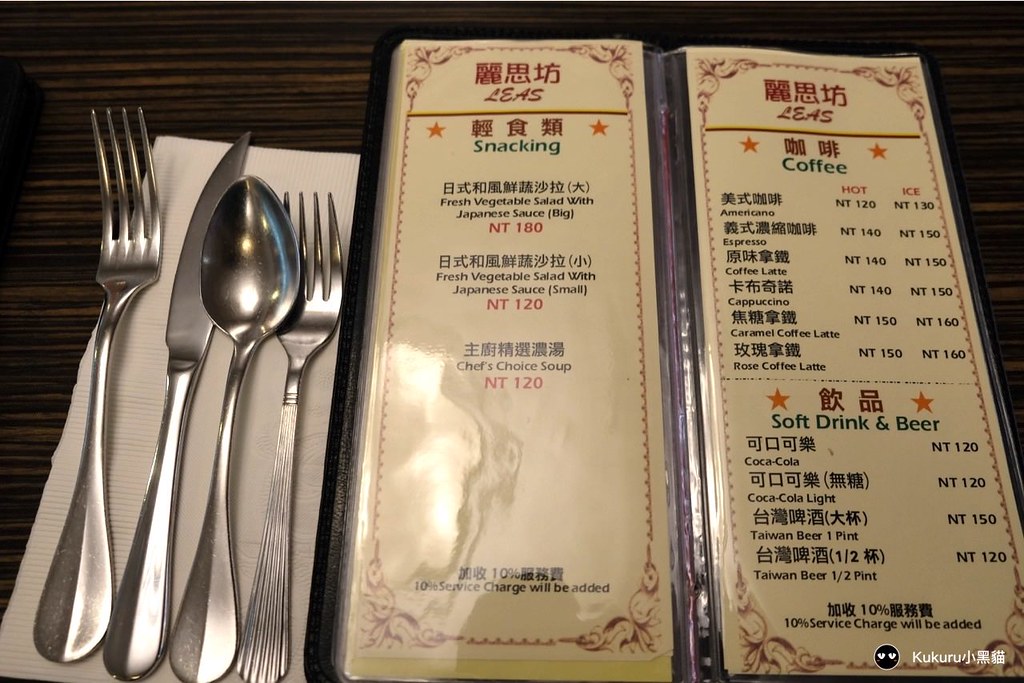The image portrays an elegantly arranged place setting and an open menu on a dark wooden table. The wood's grain, featuring both dark and light rings running horizontally from right to left, adds a rich texture to the composition.

On the left side of the image, set meticulously and angling slightly towards the upper right corner, there is a white napkin and a trio of cutlery items—all part of a matching set. The dinner fork, equipped with four tines, has a wide handle that features a central line and flares out at the end. Next to the fork is a dinner knife and a spoon, each displaying the same design characteristics. To the right of this trio is a dessert fork, distinct in its more delicate construction with four shorter tines and a handle made up of six fused strands, visibly detailed with lines meeting at a band below the tines.

On the right side of the table, an open menu predominantly in Chinese characters is displayed. The left page of the menu lists items under the heading "Snacking," written in green letters beneath red Chinese text. The listed items include "Fresh vegetable salad with Japanese sauce (big)," "Fresh vegetable salad with Japanese sauce (small)," and "Chef's choice soup." The menu notes that a 10% service charge will be added.

The right page of the menu features beverages, with sections for coffee, soft drinks, and beer. The coffee offerings include Americano, espresso, café latte, cappuccino, caramel coffee latte, and rose coffee latte. The soft drinks and beer section lists Coca-Cola, Coca-Cola Light, Taiwan beer by the pint, and Taiwan beer by the half pint, and also indicates a 10% service charge will be added. The menu is printed on a cream-colored background, bordered with an intricate red flower design engraved in each corner. Additionally, small orange stars flank the headings for coffee, soft drinks, and beer.

This sophisticated setup, combined with the meticulously detailed cutlery and ornate menu, suggests a refined dining experience.